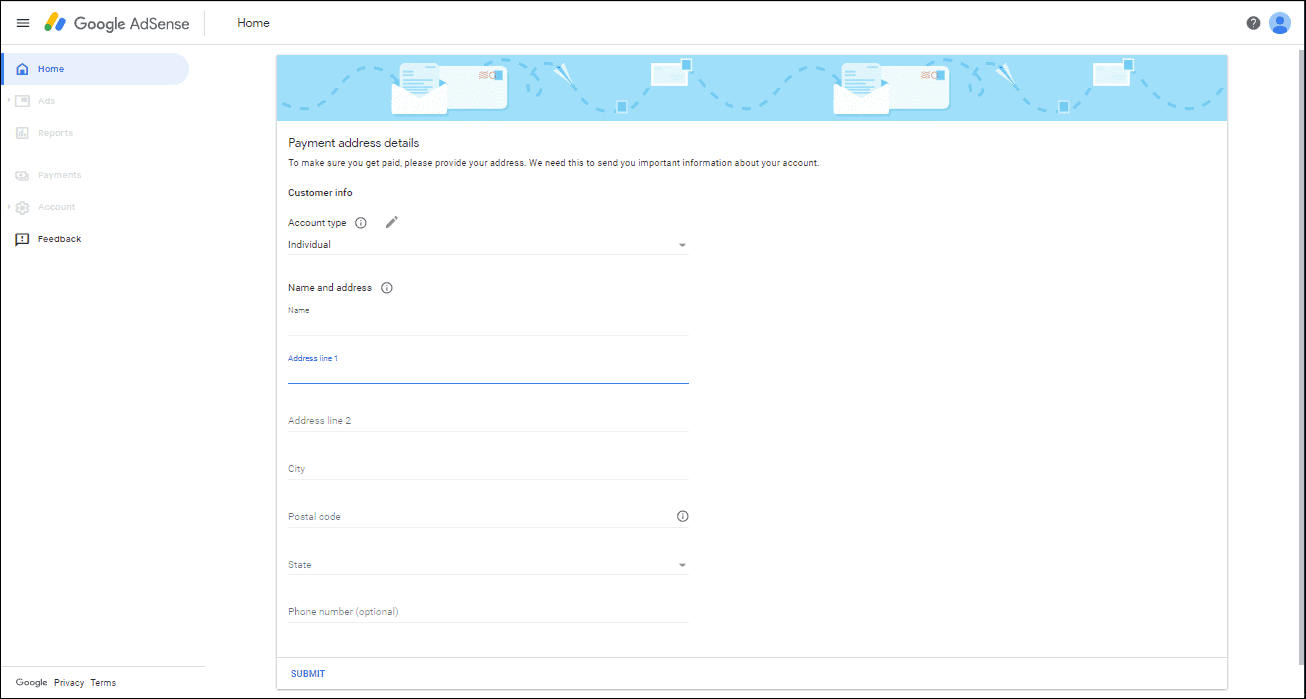The screenshot depicts a Google AdSense account interface. At the very top left, "Google AdSense" is prominently displayed, followed by the word "Home." On the far right of the screen, there is a blue circle containing a generic person icon. 

The left sidebar of the screen features a menu, with the first option labeled "Home" highlighted in blue.

The main section of the screen, on the right, is bordered by a light blue frame with envelope icons and lines, suggesting the notion of sending or mailing information. Within this section, the text "Payment Address Details" is displayed clearly, with an instruction to provide an address to ensure payment and receive important account information.

Following this, the section is labeled "Customer Information" with a subheading "Account Type," accompanied by a dropdown menu currently set to "Individual." Further down, under the section titled "Name and Address," there are several blank fields: "Name," "Address Line 1," "Address Line 2," "City," "Postal Code," and "State." Additionally, there is a field for a phone number marked as optional, which is also blank.

At the bottom of the main section is a blue "Submit" button, indicating the action to complete the form submission.